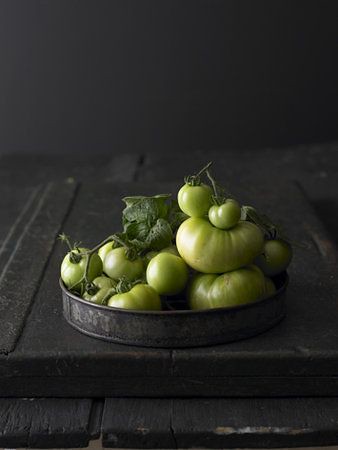This rectangular indoor photograph showcases a professional setup featuring a rustic, dark wooden table with black-stained surfaces against a backdrop of charcoal gray or black walls. Central to this scene is a vintage-looking, tarnished tin platter with a shallow wall, resembling a cake tin. This platter holds a varied collection of freshly picked green tomatoes of many sizes, from small cherry-sized ones to large heirloom types. Some tomatoes are still attached to their stems, creating a natural, slightly chaotic arrangement. The green tomatoes, with occasional leaves and stems, are piled atop one another, emphasized against the dark, monochromatic surroundings that highlight their vibrant green hues. The entire setup underscores a visual contrast meant to draw attention to the freshness and natural beauty of the tomatoes.